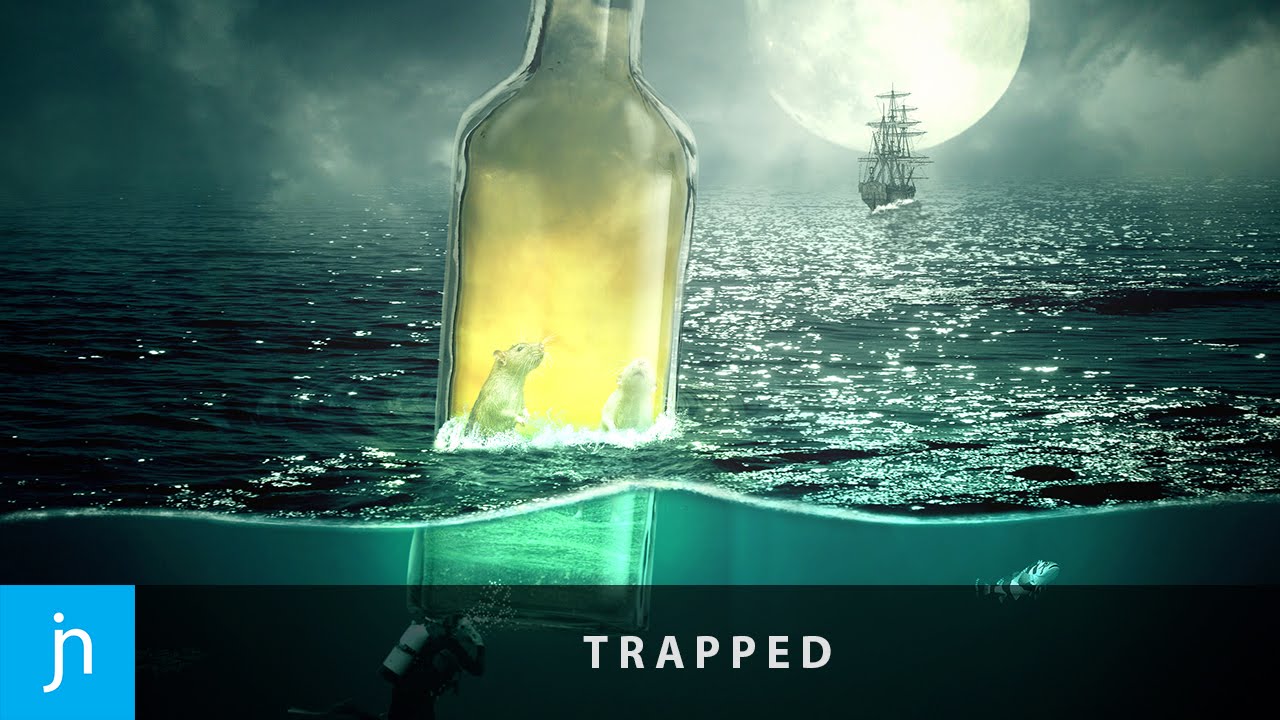In this intricately detailed artwork, possibly AI-generated or digitally edited, the scene is split between the serene surface of a calm ocean and its mysterious depths. Dominating the night sky in the upper right-hand corner, a large full moon casts a soft glow across the scene. A majestic old-fashioned wooden ship, reminiscent of a pirate vessel, sails silently in front of the moon, silhouetted against its luminous backdrop. The left side of the image is enveloped in the darkness of the open sea and night sky.

At the center of the artwork, floating near the waterline, is an old wine bottle. Inside, two small rodents, likely mice, appear to be trapped, reflecting the ominous message conveyed by the caption at the bottom of the image. This caption, “TRAPPED,” is displayed in all capital white letters on a slightly translucent dark bar overlaying the artwork. An additional blue square in the bottom left corner, possibly bearing the initials “J N,” hints at the artist’s signature or logo.

Beneath the surface, an underwater world comes into view. Directly below the floating bottle, a scuba diver hovers, adding an element of exploration and mystery. To the far right, a solitary fish swims by, adding life to the sunless aquatic expanse. The artwork is rich in nocturnal hues, with splashes of color from the dark ocean, moonlit sky, and reflective water, creating a vivid, captivating scene that encapsulates a sense of entrapment and nocturnal adventure.